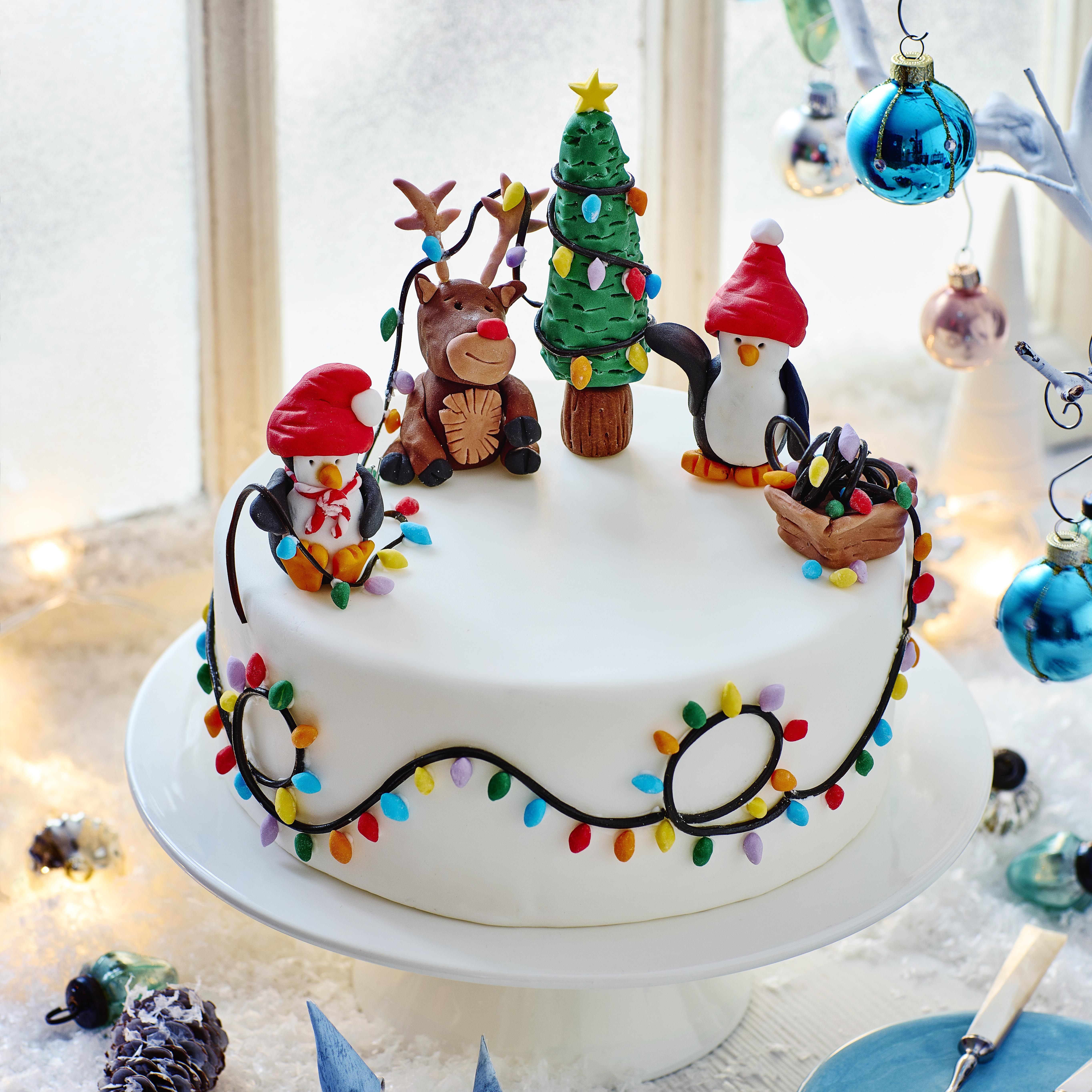This photograph captures an ornately decorated Christmas-themed cake, set on a white cake pedestal in front of a glazed glass window with three distinct panes. The cake, white with icing, is meticulously adorned to depict a charming winter scene. Colorful candy icing strings form Christmas lights, draped from a basket atop the cake and extending around the cake itself. Two penguins with red hats, a reindeer with antlers and a red nose, and a Christmas tree with a star on top are among the edible figurines made of moldable icing, each interacting with the festive lights. Surrounding the cake stand is faux powdered snow, interspersed with Christmas ornaments and acorns, enhancing the winter decor. On the table, which is well-lit, lies a blue plate accompanied by a white-handled utensil. To the right of the cake stands a white metal tree festooned with blue, silver, and pinkish ornaments, completing the festive setup.